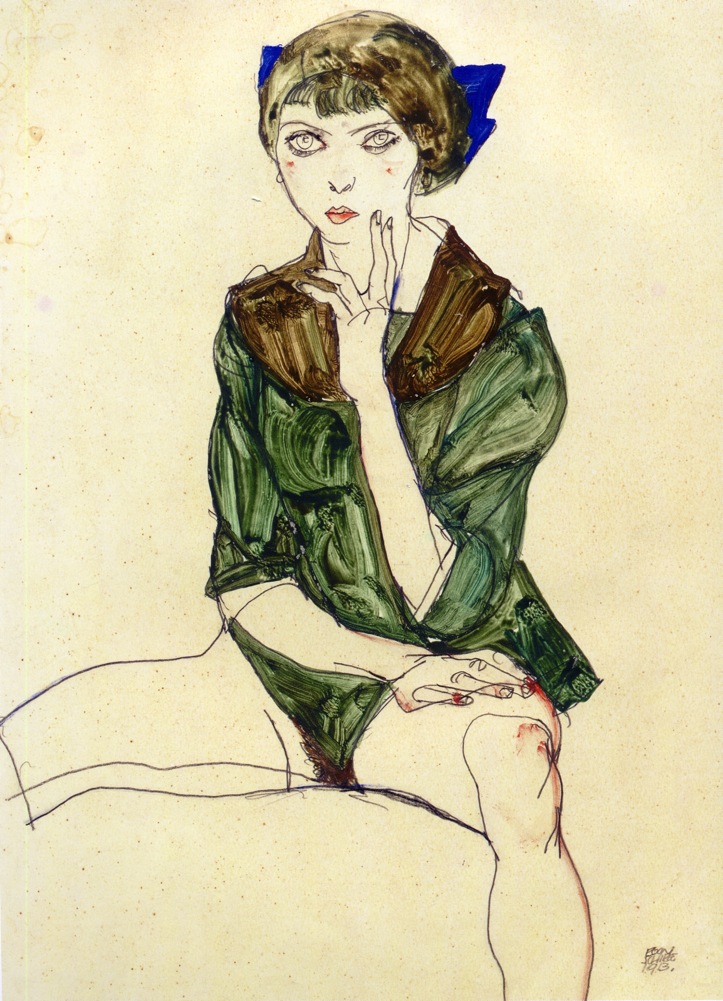The image is a detailed, hand-drawn, and colored portrait of a young woman sitting on the ground with her legs spread apart, revealing a glimpse of her groin with some pubic hair visible. The background is a dingy beige, evoking the appearance of old, aged paper. The woman has short, brownish-green hair adorned with a bright neon blue ribbon or decoration. Her face shows signs of makeup, with red spots on her cheeks and bruised-looking lips. She is seen placing her left hand thoughtfully on her face. She wears a green jacket or shirt with a distinctive brown scarf or collar. The jacket seems to have been colored perhaps with watercolor or oil paint to enhance the initial line drawing. There are also traces of blood on her hands and one leg, adding a disturbing element to her serene yet vulnerable pose.